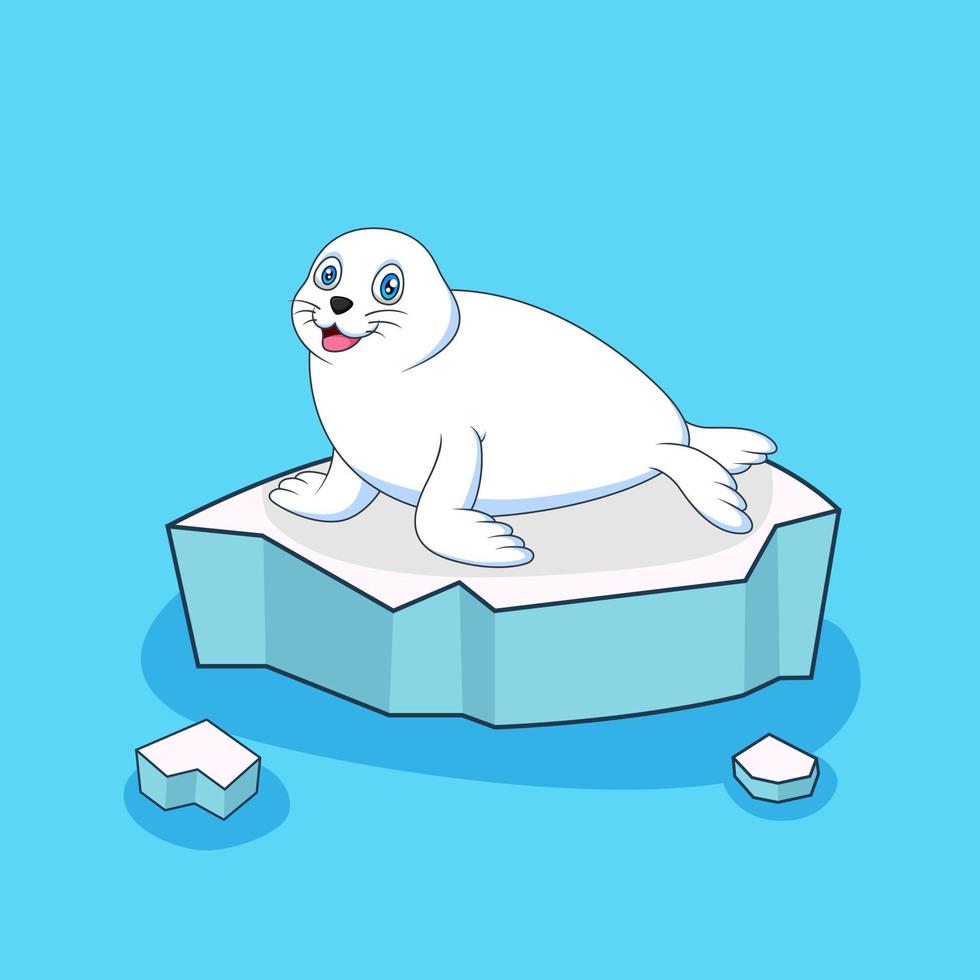This image is a detailed cartoon illustration, set against a solid light blue background. At the center of the image, there is a playful, white seal resting on a chunk of ice. The seal, outlined in black, features an elliptical body with front flippers propped up sideways and rear flippers stretched out, giving it a relaxed posture. Its smiling face, with blue oval eyes, a pink tongue, and a black nose adorned with several whiskers, is turned towards the viewer. The seal sits on a flat iceberg that is white on top with light blue sides, adding depth to the illustration. Two smaller ice chunks, similarly colored, float in the foreground, enhancing the scene’s frosty environment. The overall style of this artwork is reminiscent of children’s books or comic strips, characterized by its clear, bright colors and friendly, approachable design.